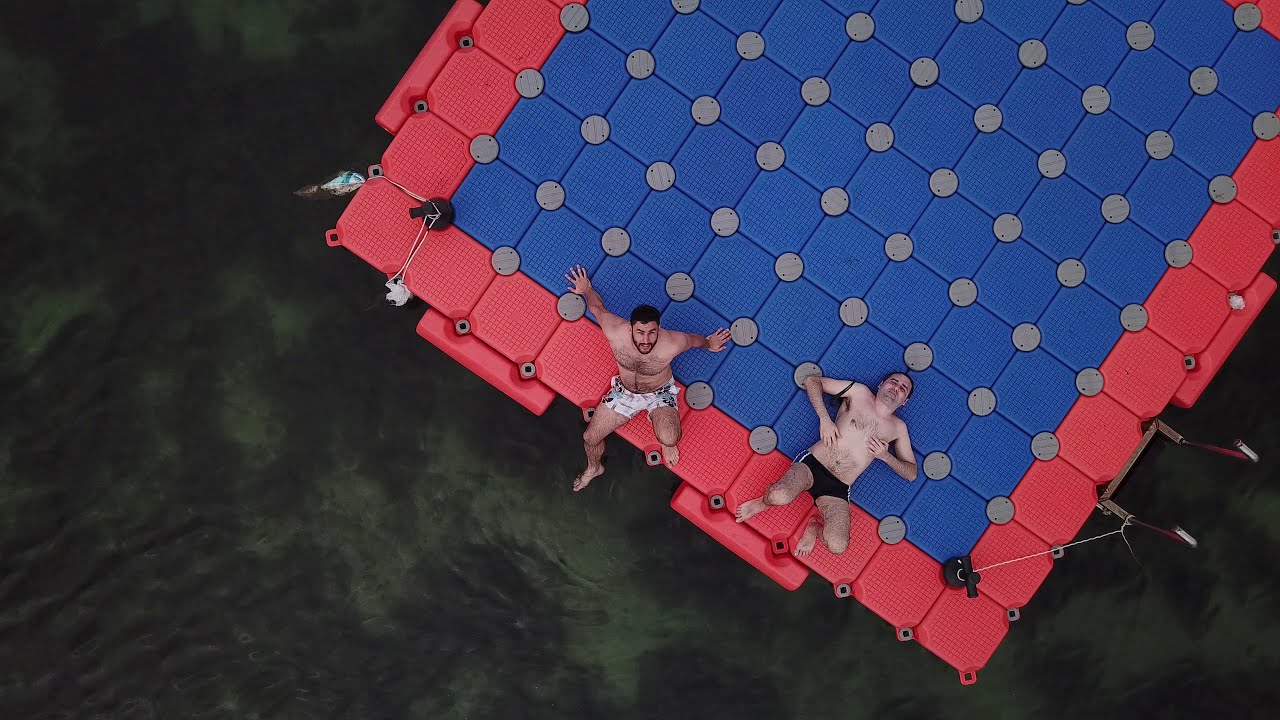This aerial image, taken from an elevation of about 20 to 30 feet, captures a vibrant dock or platform floating in murky water. The floating structure emerges from the upper right-hand corner and top edge of the frame, constructed from individual square tiles. The central portion features a blue square surrounded by a red edge, while the perimeter consists of pink squares, all interspersed with gray circles at their corners. Resting on the platform are two men in swim gear. One man is sitting with his hands back, looking directly up at the camera, wearing white shorts with black floral print, and sporting a hairy chest. The other man is lying down, dressed in black shorts with white stripes and has a black string tied around his arm. The water surrounding the platform varies in color, transitioning from a dark, deep green to an algae-like green, with subtle ripples indicating its presence.